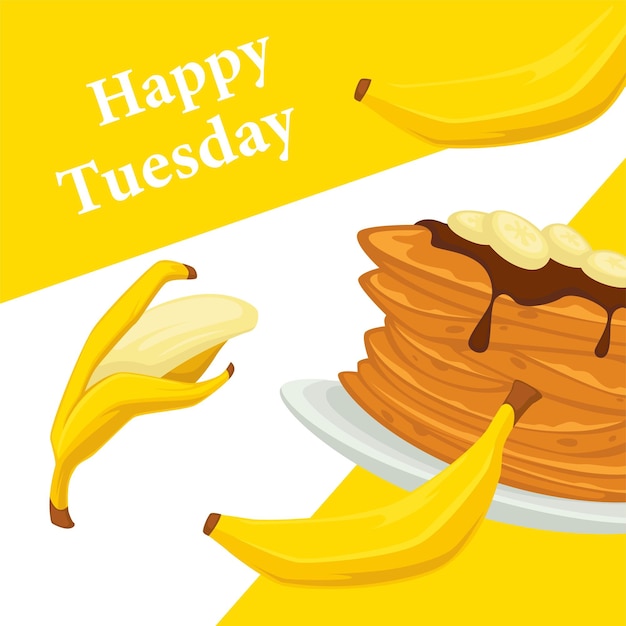This is a vibrant graphic advertisement predominantly in yellow, white, and brown tones, celebrating "Happy Tuesday." At the top, a diagonal yellow banner thicker on the left tapers to the right, with “Happy” centrally written in large white letters and “Tuesday” positioned closer to the left. The background splits into a yellow upper left corner and a yellow bottom right corner, with a white field running diagonally from right to left.

Central to the image is a white plate stacked high with approximately six banana pancakes, draped in syrup and garnished with four banana slices. Adjacent to the plate towards the right stands an unpeeled banana, featuring a pure yellow color with brown tips. 

A peeled banana, whitish yellow in hue, displays prominently in the white space, while another closed banana peeks from behind the top yellow banner, connecting this cohesive and cheerful Tuesday morning scene. The overall visual appears to be digitally rendered, adding a polished finish to the composition.